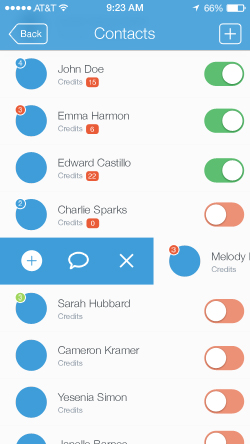The image is a screenshot taken from a smartphone, which shows a list of contacts with some additional information. The top of the phone's screen displays a blue status bar. In the top left corner, it shows the AT&T carrier logo, followed by five white circles indicating a full signal strength. Next to that, there's a Wi-Fi icon, the current time "9:23 a.m.," and a battery icon showing 66% charge.

Below the status bar, there is a navigation bar with a back arrow on the left and the word "Contacts" in the center. Under this, there is a square button with a "+" symbol in the middle, likely for adding new contacts.

The list of contacts starts with the following names along with their corresponding credits: 
- John Doe - Credits: 15
- Emma Harmon - Credits: 6
- Edward Castillo - Credits: 22
- Charlie Sparks - Credits: 0

Below these, additional names are listed: 
- Sarah Hubbard
- Cameron Kramer
- Yosania Simon
- Melody (no last name provided)

Each contact has a blue circle on the left side, some of which contain notifications. On the right side of each name, there is a toggle bar. The toggles for the first three contacts (John Doe, Emma Harmon, Edward Castillo) are turned to the right and are green, indicating they are active. The rest of the toggles, starting from Charlie Sparks, are red and turned to the left, indicating they are inactive.